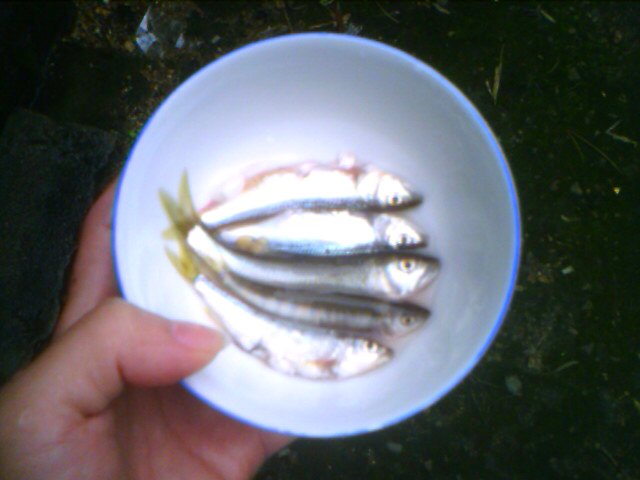This overhead photograph captures a human hand entering from the bottom left corner, with the palm and thumb visible as they hold a white bowl. The hand's thumb arches over the bowl's rim, and only parts of the pointer finger are visible underneath the bowl. The backdrop is fairly dark, revealing glimpses of green grass, sticks, rocks, and dirt scattered around. Inside the bowl are five dead minnows, laid out on their sides. The minnows have a grayish-silver hue and are aligned head to the right and tail to the left. The top two minnows have their bellies up, while the bottom three minnows lie with their backs upwards. The bowl's white interior reflects some light, adding to the overall contrast between the bright bowl and the dark, indistinct background. The fish appear fresh, with slightly open eyes, and there are no accompanying sauces or broths in the bowl.